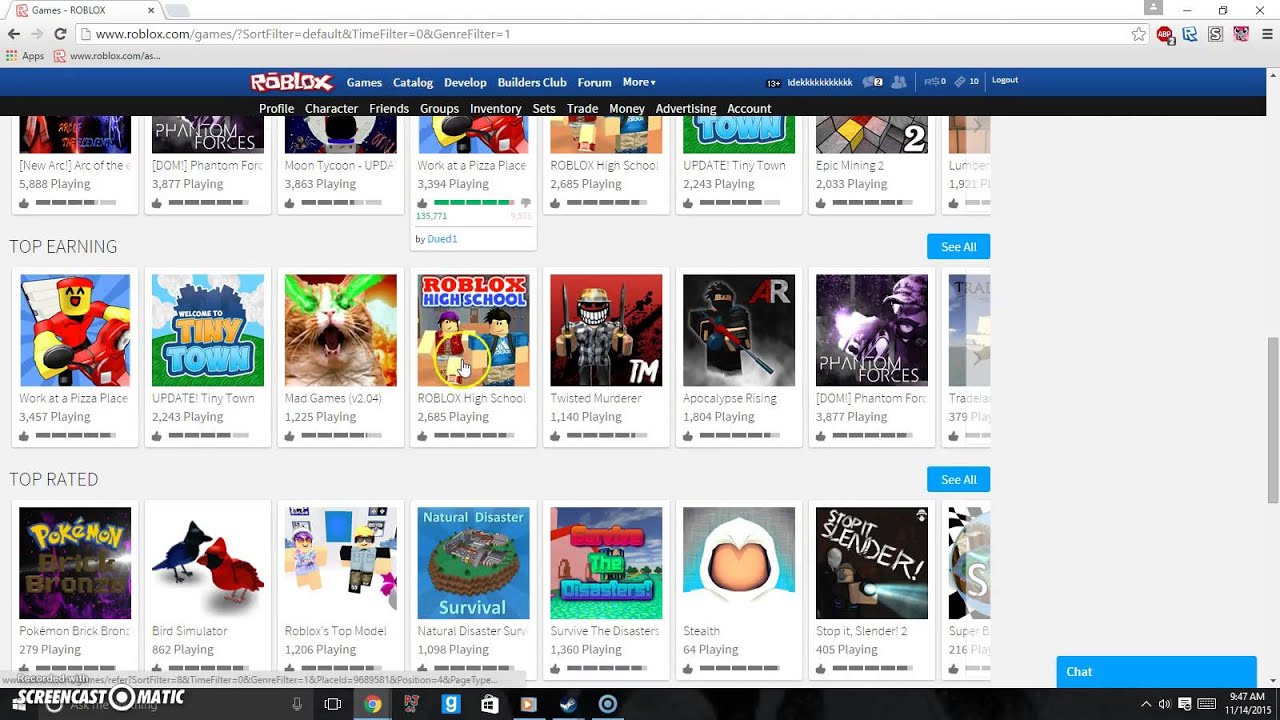Here is a detailed and cleaned-up caption for the image:

---

The screenshot displays the Roblox website open in a web browser. At the top of the window, the URL bar shows the Roblox URL. The browser tab on the top left corner features the red Roblox icon and the title "Games - Roblox." Below the URL bar, there is a gray section labeled "Apps" in the upper left corner, accompanied by the Roblox icon and URL to its right.

Further down, a dark blue navigation bar is prominently labeled with "Roblox" in red-outlined white letters. Adjacent to this title, the menu options in white text list "Games," "Catalog," "Develop," "Builders Club," "Forum," and "More," with corresponding icons for people, messages, and notifications located on the right-hand side of the navigation bar.

A thin black bar beneath this features links in white text: "Profile," "Character," "Groups," "Inventory," "Sets," "Trade," "Money," "Advertising," and "Account." Below this, the main section of the page is visible, displaying rows of game images with snippets of descriptive text. 

The top row includes partially visible game thumbnails, highlighting titles such as "New Arc" and "Arc of the," alongside gameplay statistics such as "5,888 playing" and a thumbs-up rating system. 

The second row, titled "Top Earning" in the upper left corner, is followed by a blue rectangle on the right labeled "See All." This row also showcases approximately eight or nine game images.

The final row is titled "Top Rated" on the upper left, with the first game being "Pokemon." Similarly, there is a "See All" blue button on the upper right. The bottom right corner of the page houses a blue rectangular button labeled "Chat." 

Additionally, a vertical gray scroll bar appears on the far right side of the screen. 

The bottom of the screenshot displays the Windows taskbar, where various icons are visible: "Screencast-o-Matic" in large white lettering on the left, followed by icons for a microphone, phone, Google Chrome, an illegible red icon, a blue square with a white "G," a Windows briefcase, an orange and white play button, a tool icon resembling the Steam Logo by Valve, and a white circle within another white circle. The taskbar also shows the date and time as 9:47 AM on 11-14-2015, alongside icons for a keyboard, a "Do Not Disturb" message notification, and the sound indicator showing the sound is turned on.